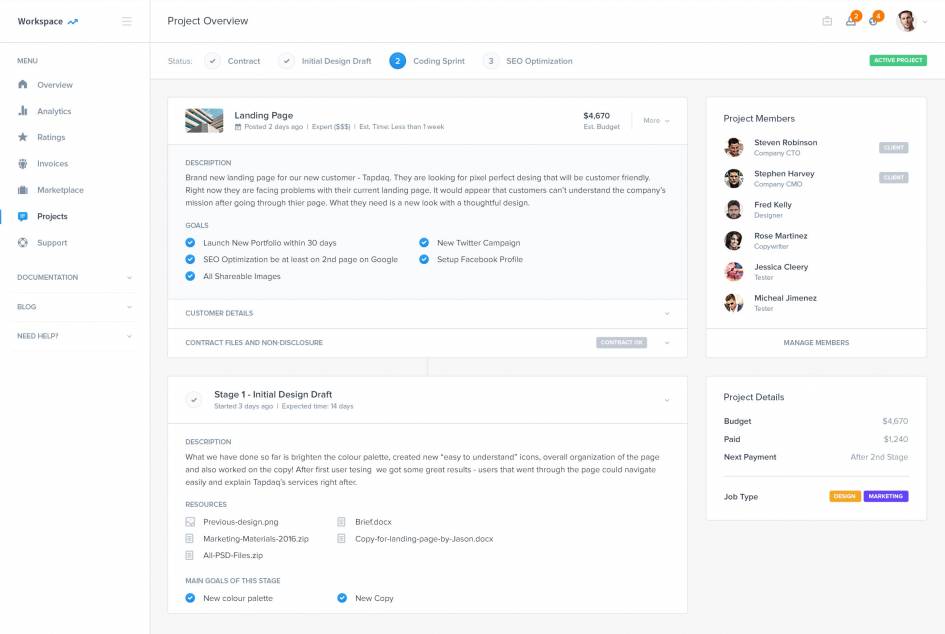**Project Management Dashboard Screenshot: Detailed Description**

The screenshot depicts a comprehensive project management dashboard titled "Project Overview," designed within a workspace environment. The dashboard offers a centralized view of the project's status and various essential elements.

**Navigation Menu:**
On the left side, there's a vertical navigation menu with the following options:
1. Overview
2. Analytics
3. Ratings
4. Invoices
5. Marketplace
6. Project Support
7. Documentation
8. Blog
9. Need Help

**Project Status:**
Below the title is a horizontal progress tracker that highlights the key stages of the project:
1. Contract
2. Initial Design Draft (highlighted with a blue circle, labeled as stage 2)
3. Coding Sprint
4. SEO Optimization

**Main Page:**
The main section showcases a project card for a "Landing Page," which was posted two days ago. The card provides a detailed description mentioning the need for a new landing page for the customer, emphasizing a pixel-perfect design that is customer-friendly. The project has a budget of $4,670. The goals outlined are:
- Launching a new portfolio within 30 days.
- Achieving SEO optimization to ensure the page is at least on the second page of Google results.
- Creating all shareable images.
- Developing a new Twitter campaign and setting up a Facebook profile.

Additionally, there's a placeholder section for customer details and contract files.

**Project Members:**
On the right side, the dashboard panel lists the project members, including their roles and small profile pictures:
- Steve Robinson - Company CTO
- Stephen Harvey - Company CMO
- Fred Kelly - Designer
- Rose Martinez - Copywriter
- Jessica Cleary - Tester
- Michael Jimenez - Tester

There are options available to manage the members in this panel.

**Overall Organization:**
The dashboard is meticulously organized, providing a clear and comprehensive overview of the project's status, the members involved, and the financial details, ensuring that all aspects of the project are easily accessible and manageable.